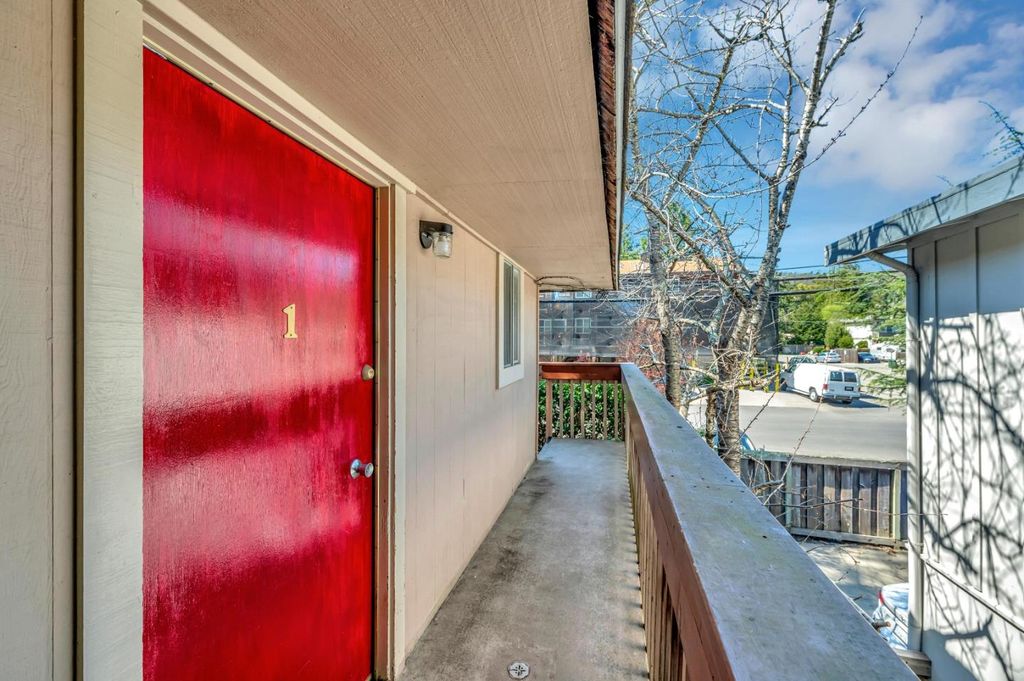The photograph captures the entrance to a building as seen from an external balcony. The camera is positioned on the balcony, providing a forward-looking perspective. To the right, a sturdy railing runs parallel to the edge of the balcony and makes a sharp 90-degree turn to the left towards the back of the frame. On the left-hand side at the very front of the image stands a vivid red exterior door adorned with a metal handle and the gold numeral "1." The building's siding features a light tan to white color, complementing the bright door. An overhang extends from the ceiling above, sheltering the balcony area.